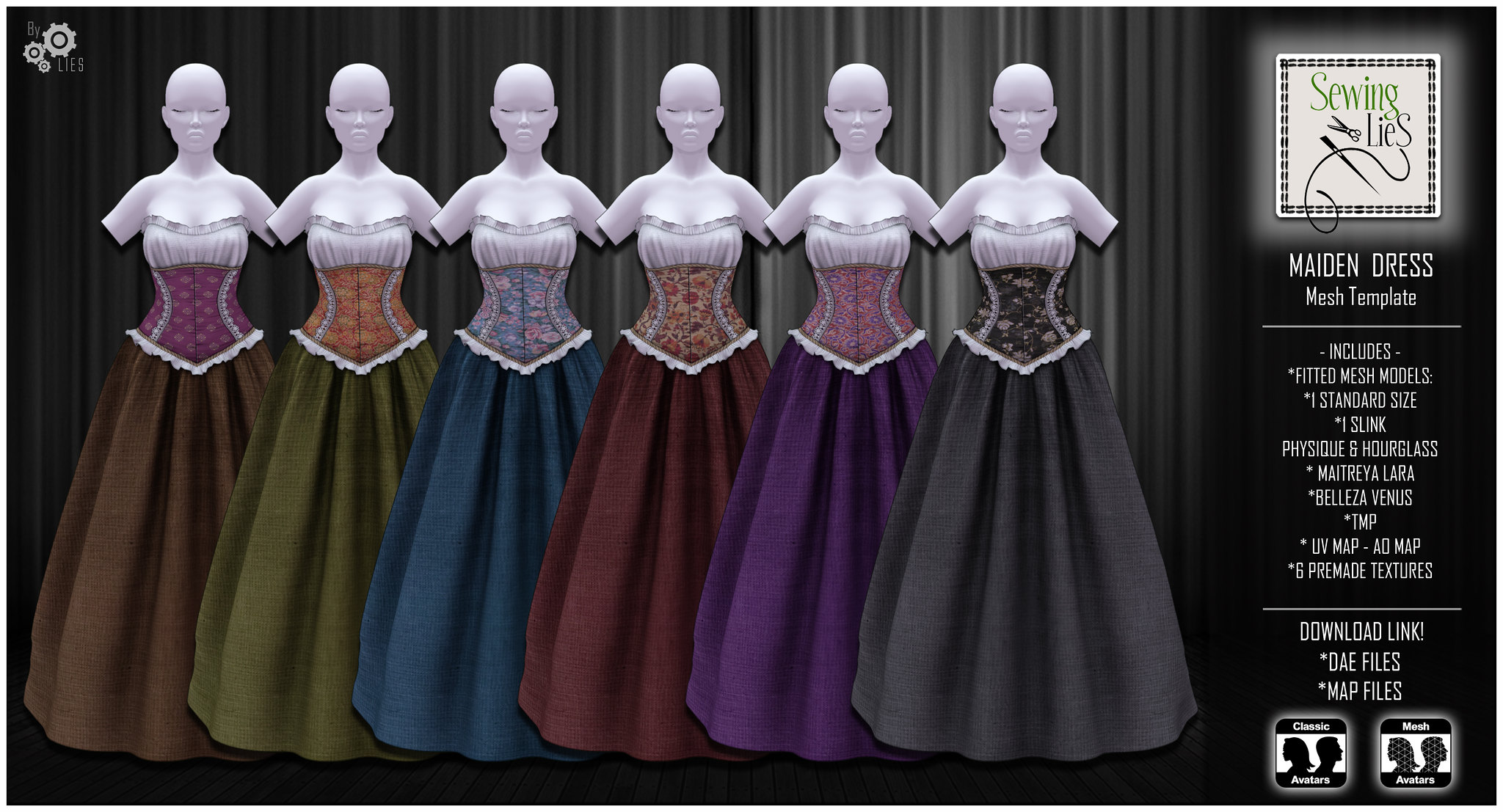In a detailed product image, a backdrop of gray curtains sets the stage for six graphically designed mannequins, each devoid of arms and sporting long, Renaissance-style dresses. The mannequins, characterized by their closed eyes and bald, white heads, display dresses that fit snugly on the chest and belly before flaring out. The dresses, identical in style but varied in color, are arranged from left to right as follows: a burgundy and brown dress, an orange and green dress, a purple and navy blue dress, a yellow and gold dress, a light and dark purple dress, and a black and white dress. Each mannequin's dress features a corset-like top. To the right of the mannequins, a text box reads: “Sewing Lies, Made in Dress, Mesh Template Includes, Fitted Mesh Model, One Standard Size, One Slink Physique and Hourglass, Matreya Lara, Beliza, Venus, TMP, UV Map, AD Map, G Pre-Made Texture, Download Link, DAE Files, and MAE Files, Classic Avatars, Mesh Avatar.” The comprehensive details suggest this image is promoting a digital pattern for making these elaborate “maiden dresses.”